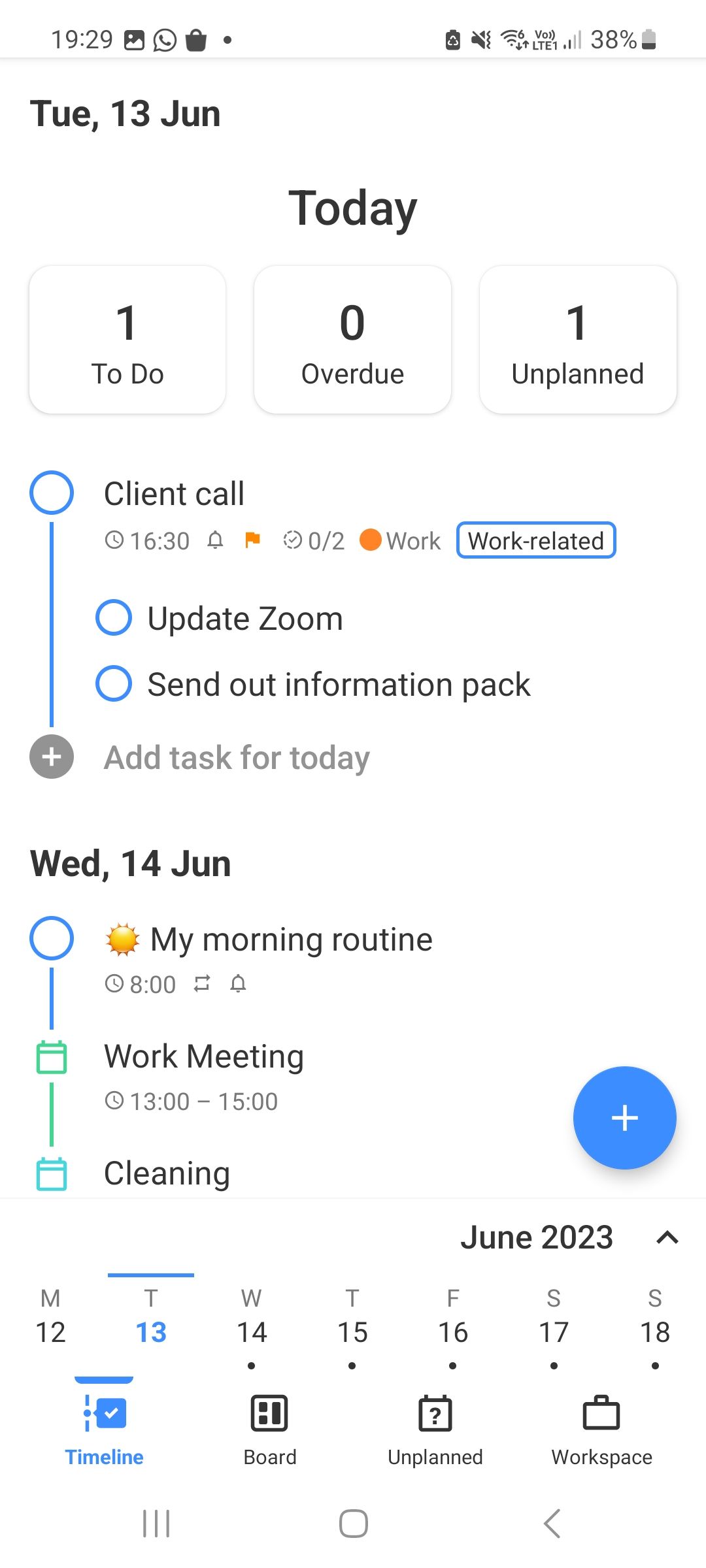Screenshot of a smartphone screen showcasing various app icons and status indicators. In the top left corner, the time reads 19:29 in 24-hour format. Immediately next to it are icons for a picture (likely Facebook Messenger), a shopping bag, and a dot. 

The status bar indicates that Battery Saver mode is activated, the phone is on silent mode, Wi-Fi signal strength is at full bars, cellular signal strength is at 2 out of 4 bars, and the battery level is at 30%.

Below the status bar, today's date is displayed as Tuesday, 13th of June. The planner section reveals one pending task under "To Do," with zero overdue items and one unplanned activity. There's a scheduled client call at 16:30, labeled with an orange tag for work. The related tasks are "Update Zoom" and "Send out information pack." There is also an option to add a new task, indicated by a gray circle.

For the following day, Wednesday, 14th of June, the schedule includes a morning routine starting at 08:00, a work meeting from 13:00 to 15:00, and cleaning activities marked with a blue circle. 

The calendar at the bottom shows the current week of June 2023, listing the days from Monday (12th) to Sunday (18th). The interface includes sections for "Timeline," "Board," "Unplanned," and "Workspace," reflecting various organizational tools and features available.